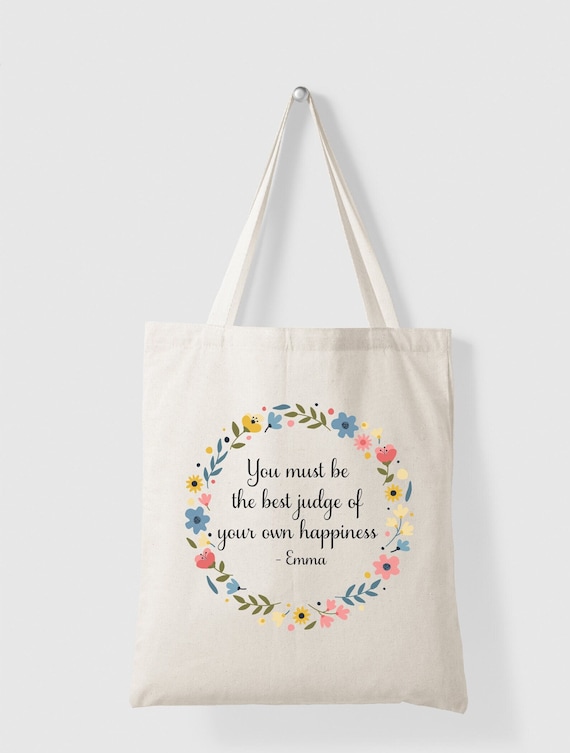In the image, we see a charming off-white cloth handbag, reminiscent of a grocery tote bag. The bag features handles long enough to be carried over the forearm, shoulder, or by hand and is hanging from a hook on a white wall. The handbag showcases a decorative circular wreath of pastel-colored flowers in yellow, pink, and blue, interspersed with little green leaves and a couple of hearts. Inside the floral wreath, cursive text reads, "You must be the best judge of your own happiness," signed with "Emma" beneath. The bag is rectangular and vertically upright, emitting a simple yet endearing aesthetic, perfect for casual everyday use.